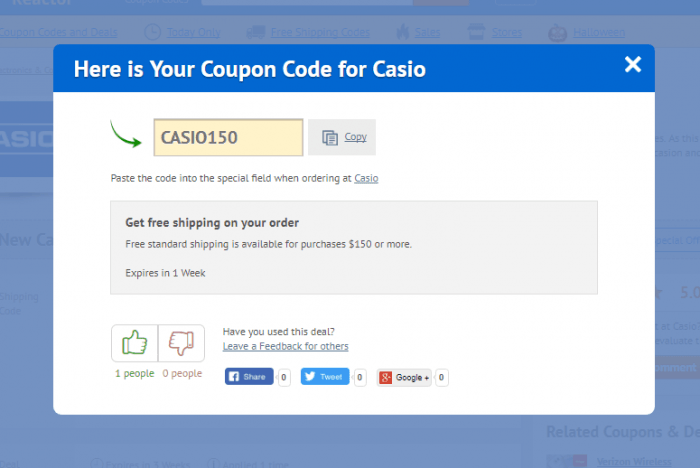The image depicts a pop-up window in the foreground, obscuring most of the background, which is grayed out and indistinct. The pop-up is a prompt box designed to offer a coupon code for Casio products. The box features a blue rectangle across the top with a white 'X' in the upper right corner, allowing the user to close the pop-up. The text in this blue section is white and reads, "Here is your coupon code for Casio."

In the center of the window, there's a green arrow pointing to a prominent yellow box containing the coupon code "CASIO150". To the right of this box is an icon depicting two overlapping pieces of paper and the word "COPY," indicating that clicking it will copy the coupon code for easy pasting during checkout.

Additional instructions below the code inform users to paste the code into the designated field when ordering from Casio. There is an underlined segment, presumably a hyperlink, that redirects users to the Casio website. Beneath these instructions, another gray box informs users that free standard shipping is available for orders of $150 or more, with the offer expiring in one week.

At the bottom of the pop-up, a green thumbs-up icon and a red thumbs-down icon show that one person has given positive feedback, while nobody has indicated a negative response. The pop-up encourages users to leave feedback if they've used the coupon code. Social media sharing options are also available, with icons for Facebook (share 0), Twitter/X (tweet 0), and Google Plus (0), indicating no social media engagement thus far.